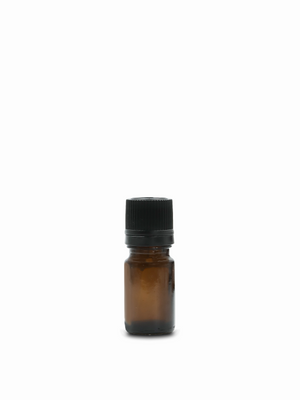The image depicts a small, dark brown glass vial with a black ridged cap, set against a plain white background. The vial is approximately two inches tall, with the cap constituting about two-thirds of the vial's total height, suggesting the cap is around one inch tall. The bottom of the vial appears to be darker than the middle section, giving the impression of it being slightly brown-black. The glass is unmarked, and the vial itself appears empty, though it is commonly used for containing essential oils or other liquids. The cap is designed for easy gripping and twisting, likely featuring a stopper. The minimalistic setting of the image emphasizes the simplicity and potential utility of the vial.